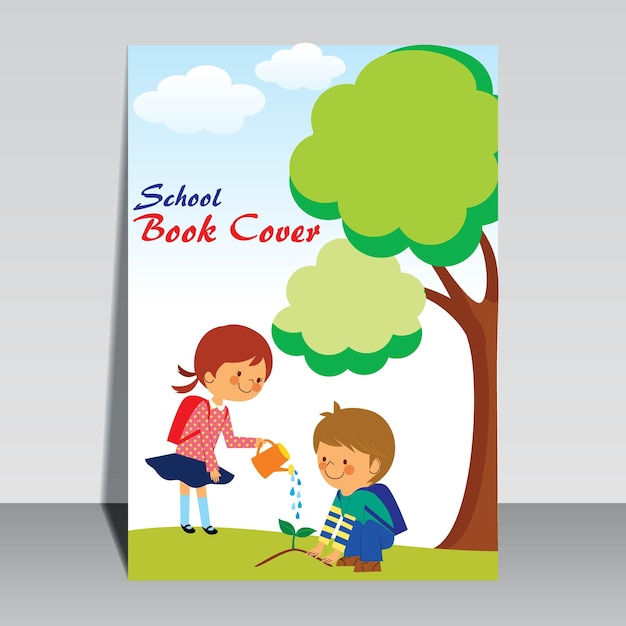The image is a color photograph in a square format, depicting a book cover or a card standing vertically on a gray tabletop, leaned against a lighter gray wall. The card features simple, animated illustrations with a focus on educational themes.

On the right side of the card, there is a brown tree trunk with light green leaves extending to the left and forming two large tufts of green foliage at the top. The backdrop includes a blue sky with white clouds. Prominently displayed at the top left portion of the card are the words "school" in blue and "book cover" in red.

At the bottom of the card, two children are depicted engaging in gardening on green grass. On the left, a young girl with red hair and a red backpack is watering a small two-leaf plant with an orange pitcher. She is dressed in a pink polka-dotted top, a blue skirt, light blue socks, and dark blue shoes. Kneeling to the right of the plant is a young boy with brown hair, smiling as he looks at the plant. He is wearing a green shirt with blue and yellow sleeves, blue pants, brown shoes, and a blue backpack. 

The overall style of the image blends realistic color photography with illustrative elements, resulting in a vibrant and engaging visual experience.